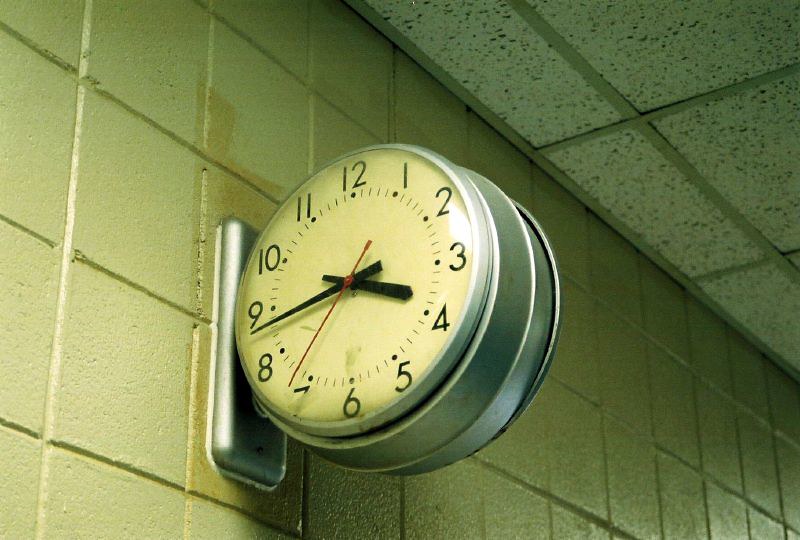This horizontal photograph captures a classic school clock, double-faced and securely mounted to a wall in an aluminum or stainless steel frame. The backdrop features greenish-colored cinder block walls arranged in a square pattern, complementing the institutional setting. Overhead, a drop ceiling with gray metal supports forms a grid, characteristic of many educational buildings. The clock's face is noticeably yellowed with age, bearing black hour and minute hands, alongside a distinct red second hand. It is affixed to the wall on a vertical rectangular metal mount, displaying the time as 3:43.